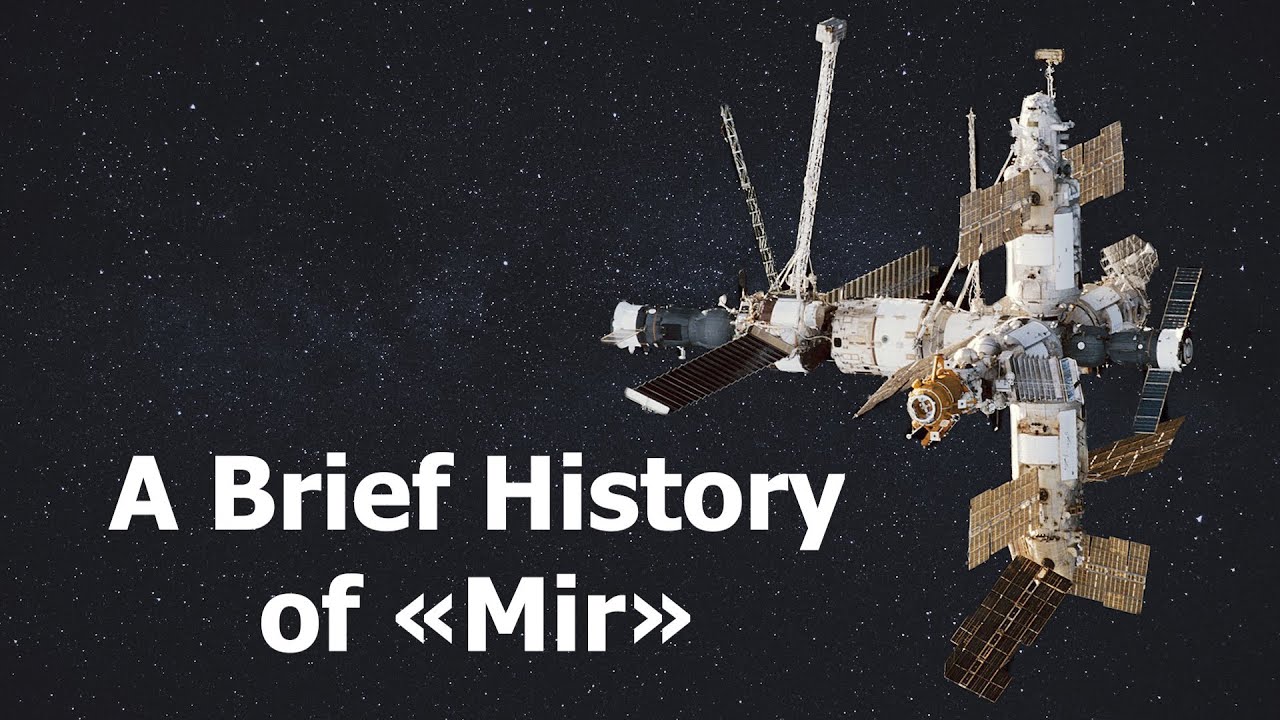This photograph features the historic Russian space station, Mir, against the vast backdrop of space. To the left of the image, large white text reads "A Brief History of Mir," with 'MIR' enclosed by outward-pointing arrows. Mir occupies the right third of the image and showcases an intricate assembly of antennas, solar panels, ladders, and electronic instruments. The space station, displaying a somewhat aged appearance with white and rust-colored sections, also includes gold and black elements—particularly the solar panels. The setting is a stark black sky dotted with white stars, highlighting the station’s striking silhouette, which resembles a sideways T shape spanning almost the entire height of the image.